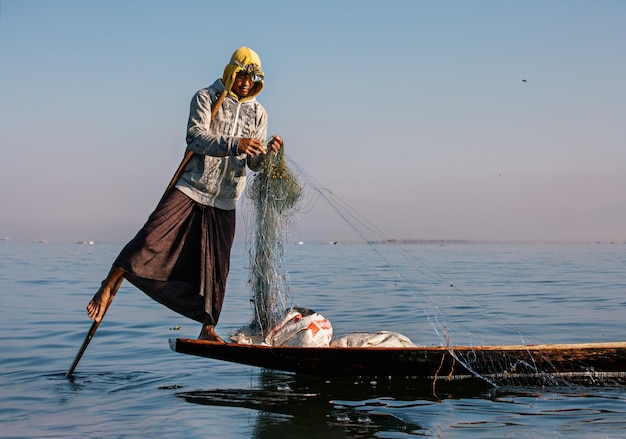In this detailed outdoor image, taken during either sunrise or sunset on a vast ocean, a man is standing on a small wooden boat. He appears to be from Southeast Asia, dressed in a dark reddish-brown cloth wrapped around his legs, a jacket, and a yellow hood to protect himself from the sun. Balancing precariously with one foot on the boat and the other wrapped around a stick that extends into the water, he works to untangle and manage a fishing net, seemingly in the midst of catching fish. Additional items, possibly bags, are situated toward the middle to the left side of the boat, suggesting the preparation or culmination of a day's labor. The serene setting highlights the beginning or end of a hardworking day on the water.